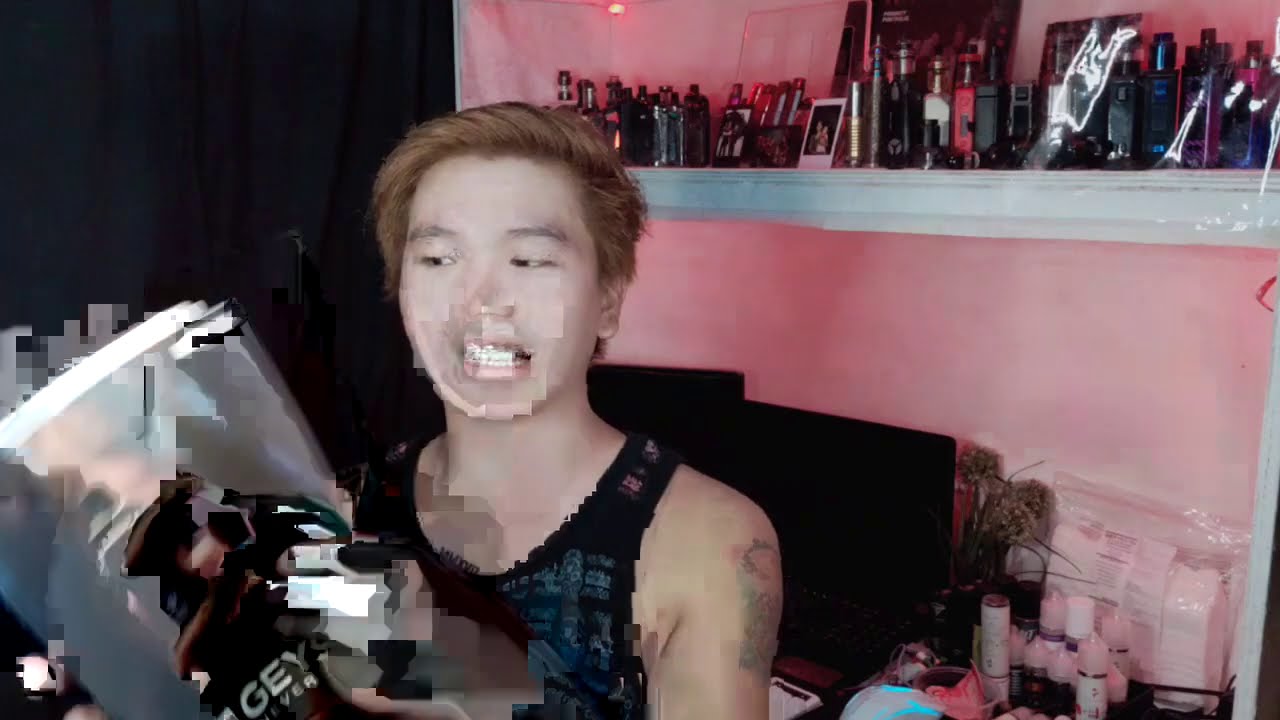The image is a screenshot from a video call, featuring a young Asian man with medium-length, auburn or ginger hair and white skin. He is sitting in the center, gritting his teeth and holding either a book or a magazine. He is dressed in a black sleeveless tank top that reveals a tattoo on his left arm. The background is a pink wall with a shelf containing various knickknacks, cosmetics, and small bottles or tubes. Below this shelf, there are two black computer screens and additional objects on a table. The image has a filter that creates a pixelated effect, particularly around the man's lower body, which gradually becomes clearer towards the top.